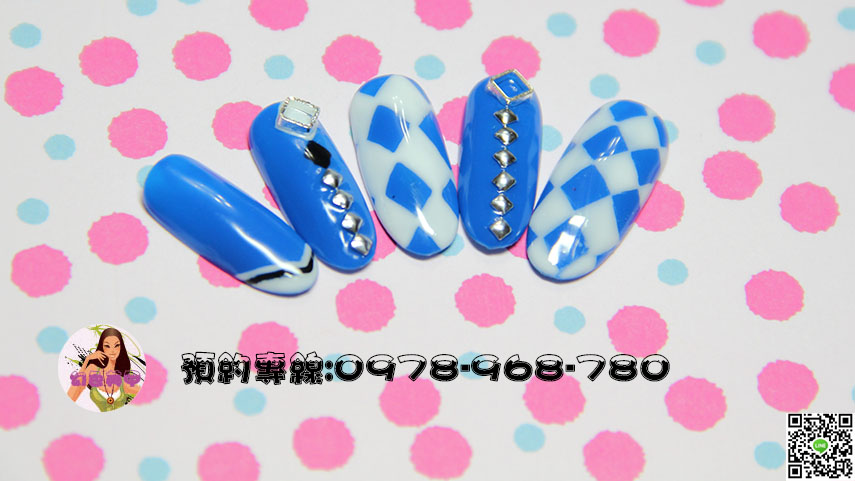The image is a colorful advertisement for fake fingernail designs, set against an off-white background adorned with large pink polka dots and smaller blue dots randomly scattered. Prominently featured in the center are five distinct blue fingernail tips, each showcasing unique patterns. From left to right: the first nail is mostly blue with a white base and a small black checkmark-like design; the second nail has a blue background with a prominent diamond shape in black and smaller silver diamond shapes; the third nail features a blue diamond pattern on a white background; the fourth nail has silver diamond-like shapes on a blue background; and the fifth nail mirrors the third with a similar blue and white diamond pattern. 

To the left of these nail designs is an illustration of a young woman with her face resting against her right hand, wearing a green blouse and a white under-top, and adorned with a necklace. Some purple Asian characters overlay her image. Below the nails is a stylized string of Asian characters alongside the phone number 0978-968-780, written in bold black font transitioning to white at the top. On the bottom right corner of the image is a QR code with a small green circular icon in the center. The background and elements converge to form an engaging and detailed promotional material.